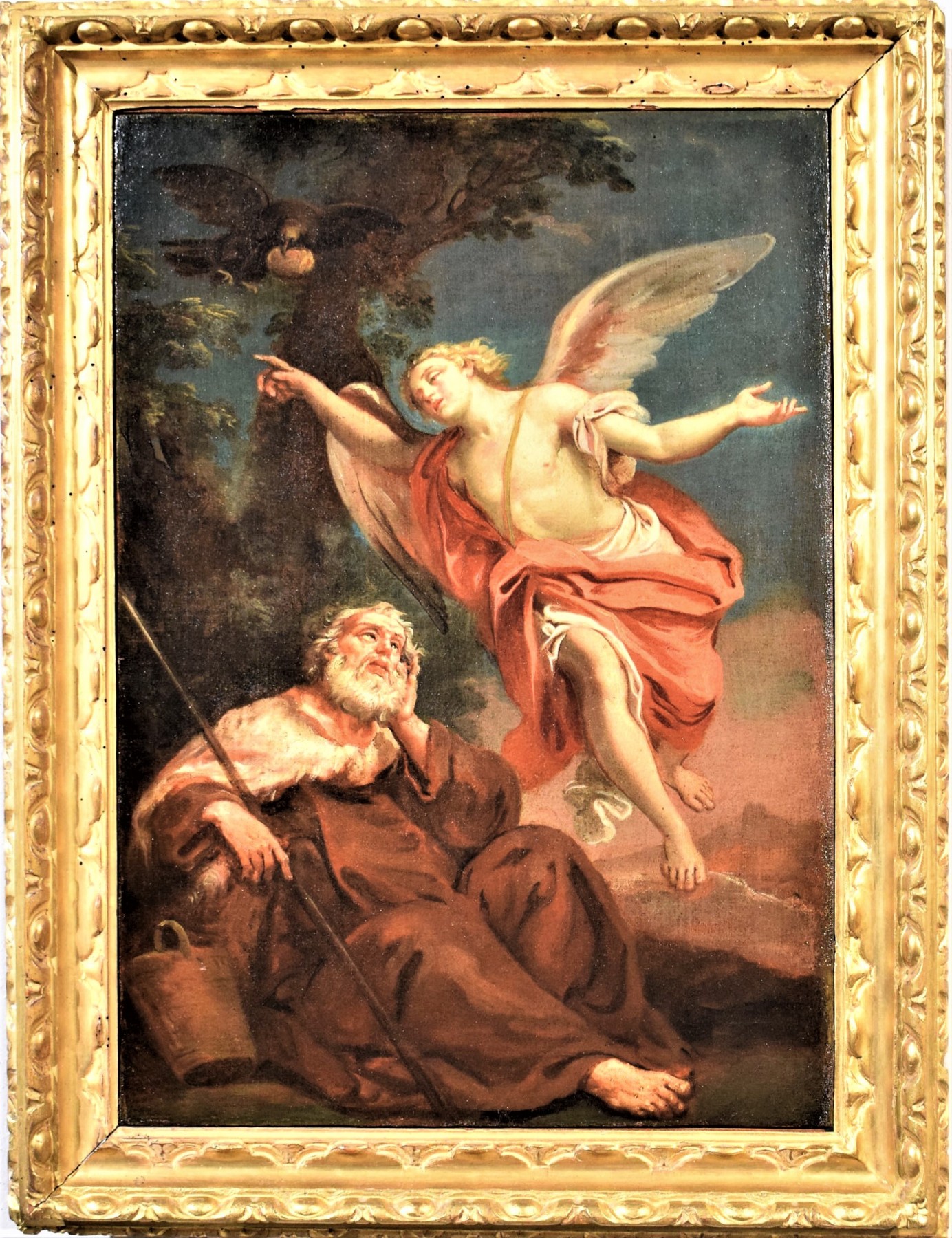The image depicts a Renaissance-era oil painting, housed in an intricately carved, golden-gilded wooden frame. At the center of this religious-themed artwork is an older man with a white beard, dressed in brown robes and sitting barefoot against a dark-colored tree. He holds a walking stick in one hand, and a small pouch lies on the ground beside him. Hovering over the man is a large angel, bare-chested but draped in red and white robes, with wings outstretched. In the upper left corner of the scene, a black bird, likely a crow, holds a piece of bread in its beak. The tree behind the man displays a single piece of fruit hanging from one of its branches. The rich details and the timeless elements of the composition highlight its Renaissance inspiration.